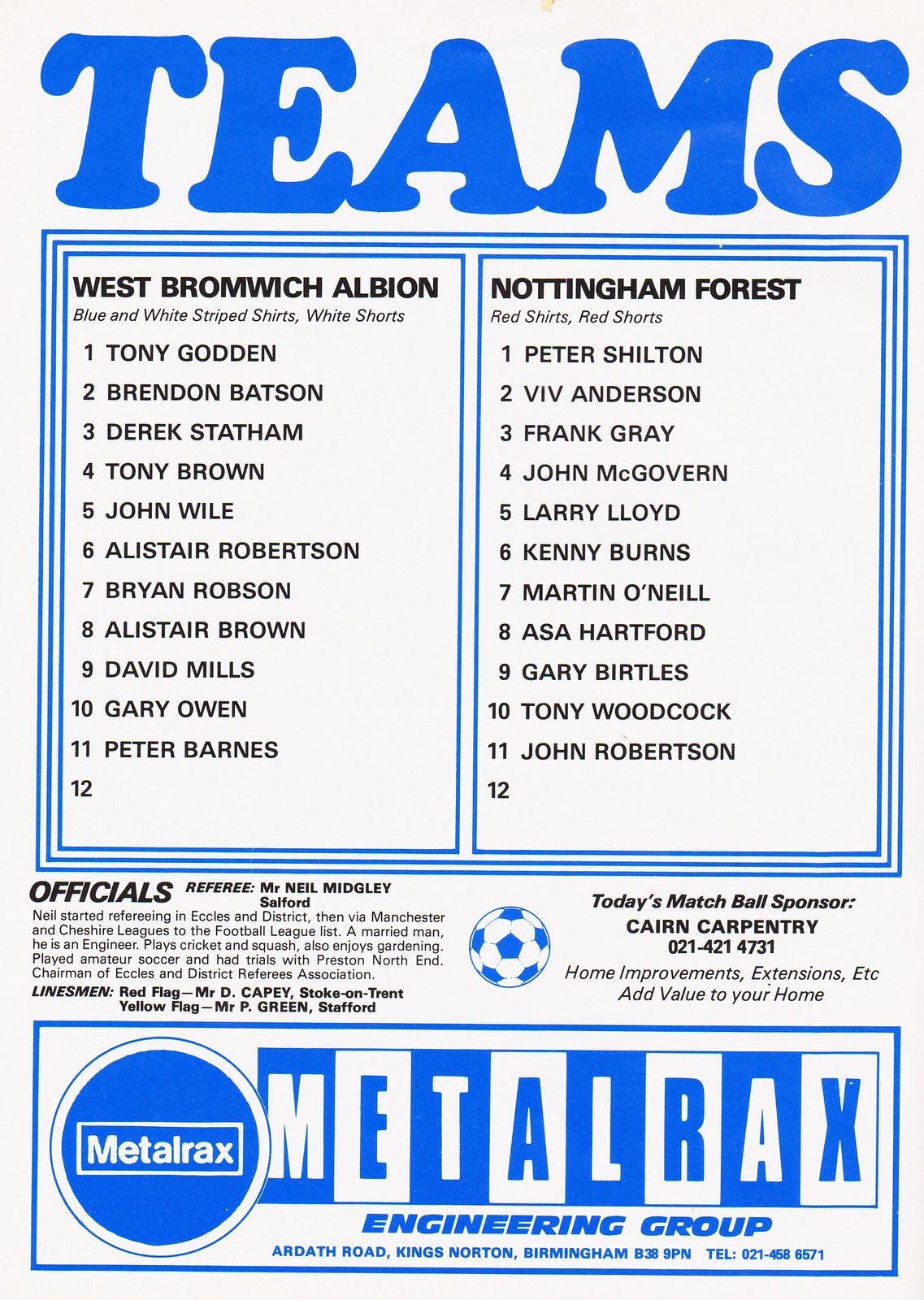The image features a white poster with bold blue and black lettering at the top, prominently displaying the word "TEAMS." Beneath this heading, two white squares list the names of 11 players each for two soccer teams. The left column, titled "West Bromwich Albion," showcases players in blue and white striped shirts paired with white shorts. The right column, labeled "Nottingham Forest," lists players donning red shirts and red shorts. 

Enclosed within a blue triple border, these columns stand out distinctly. Below the players' names, the section marked "OFFICIALS" provides the name of the match official, Mr. Neil Migley. Adjacent to it, the text reads "Today's match sponsor: Taron Carpentry," accompanied by a small image of a blue and white soccer ball. 

At the bottom of the poster, an advertisement for "Metal Racks" by the Metal Racks Engineering Group in Birmingham, England is featured. This ad uses alternating blue and white boxes with corresponding white and blue text, further accentuating the poster's overall design.